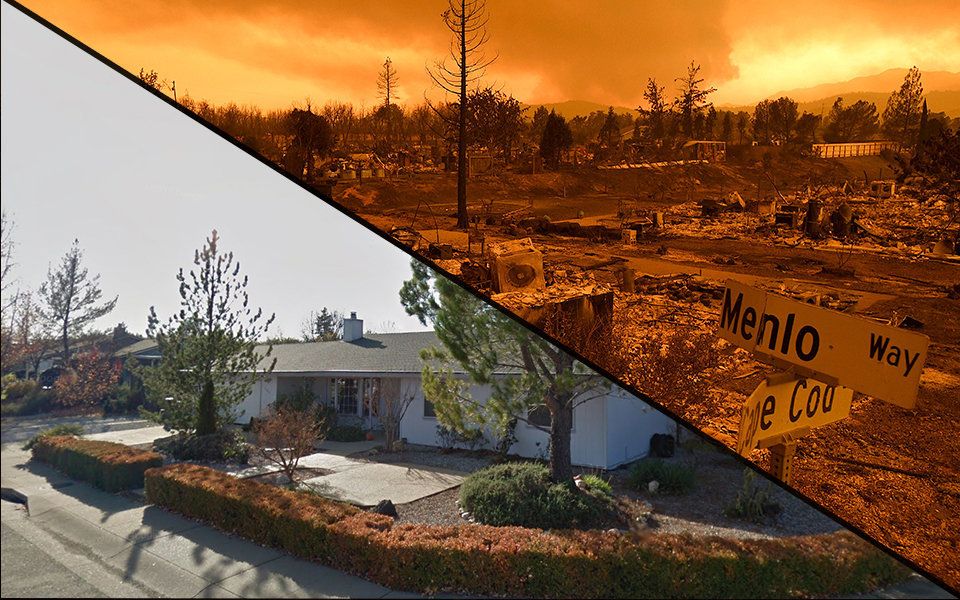This split photograph powerfully contrasts a neighborhood before and after a devastating fire. The bottom left section of the image showcases a serene, well-kept house with a green roof and white walls, complemented by glass windows, a chimney, and a front patio adorned with bushes. The front yard is meticulously landscaped with gravel, framed by trees and bushes, and includes a clearly visible driveway with other neighboring homes. In stark contrast, the top right section depicts the aftermath of the fire on Menlino Way and Cape Cod. Here, an eerie, orange-hued haze blankets the scene, and only burnt tree trunks and piles of ash and rubble remain. The devastation is evident in the barren, charred landscape where the once orderly neighborhood stood, hinting at a recent disaster that has left everything in ruins, with burnt trees and a bent sign marking the spot of destruction.